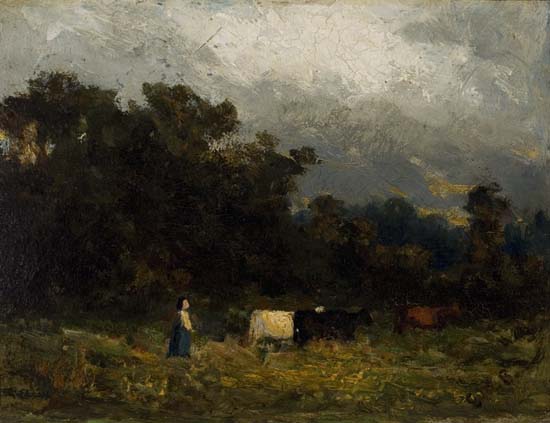This artwork, possibly an oil painting with a slightly impressionistic style, captures a somber, rural scene under a gray sky with hints of white. The setting comprises a dark, open grassy field, interspersed with patches of yellow. A dense tree line or bush, appearing almost black with splashes of brown and dark green, contrasts against the gloomy backdrop. In the foreground, a female figure with black hair and light skin stands, wearing a yellow shirt and a blue skirt. She observes three cows nearby: one predominantly white with black patches, a second all black, and a third all brown, blending into the untamed, brush-stroked landscape. This idyllic scene evokes the tranquility and simplicity of pastoral life, framed by tall, dark green trees.